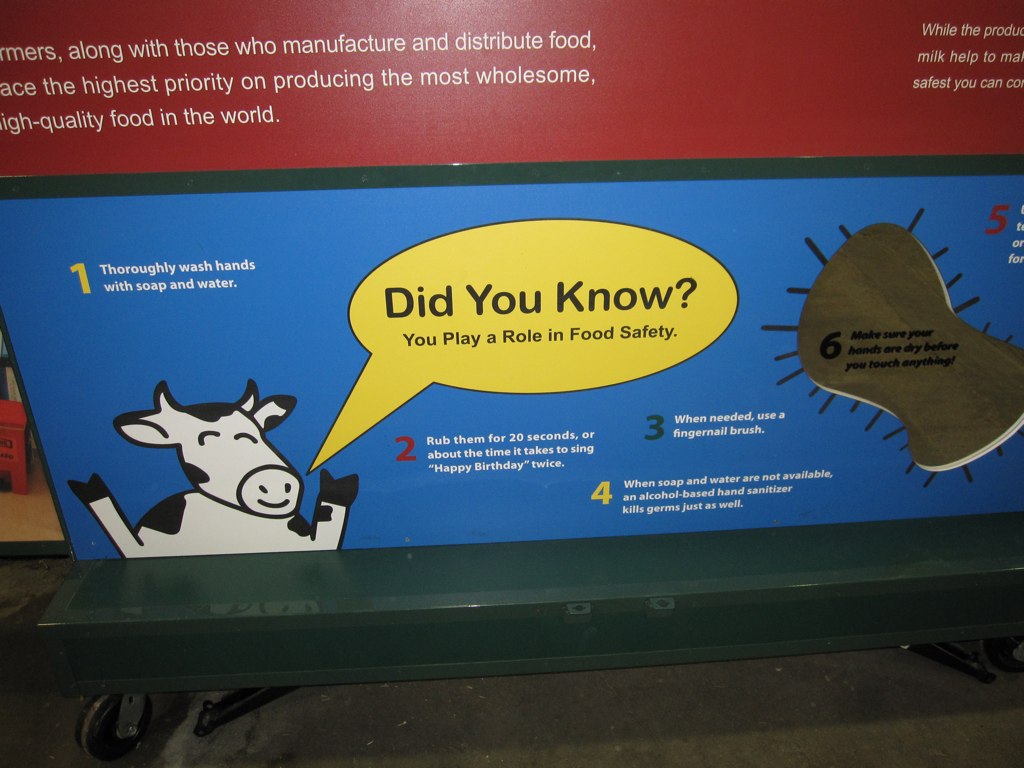The image features a detailed food safety educational poster mounted on a low-lying green cart equipped with wheels, suggesting it is designed for mobility. The setting appears to be outdoors. The central focal point of the image is the poster, which is divided into a red top section, followed by a blue rectangle separated by a black line.

At the very top in the maroon-colored section, the poster reads: "Farmers, along with those who manufacture and distribute food, embrace the highest priority in producing the most wholesome, high-quality food in the world." 

Below this, within the blue section, the poster provides specific handwashing guidelines, emphasized by cartoon graphics and colorful numbering:

1. A white number on a blue background instructs to "thoroughly wash your hands with soap and water."
2. Adjacent to this, a cartoon cow with a yellow speech bubble reads: "Did you know you play a role in food safety?"
3. The number two in red indicates to "Rub them together for 20 seconds, or about the time it takes to sing 'Happy Birthday' twice."
4. A black number three advises, "When needed, use a fingernail brush."
5. The number four in yellow details, "When soap and water are not available, use an alcohol-based hand sanitizer which kills germs just as well."

While parts of the poster’s far right are cut off, the visible portion includes an image resembling a bacterium with the number six, which likely reads: "Make sure your hands are dry before you touch anything."

The colors visible in the image include maroon, gray, black, green, blue, yellow, white, and red, contributing to the overall informative and engaging nature of the poster.